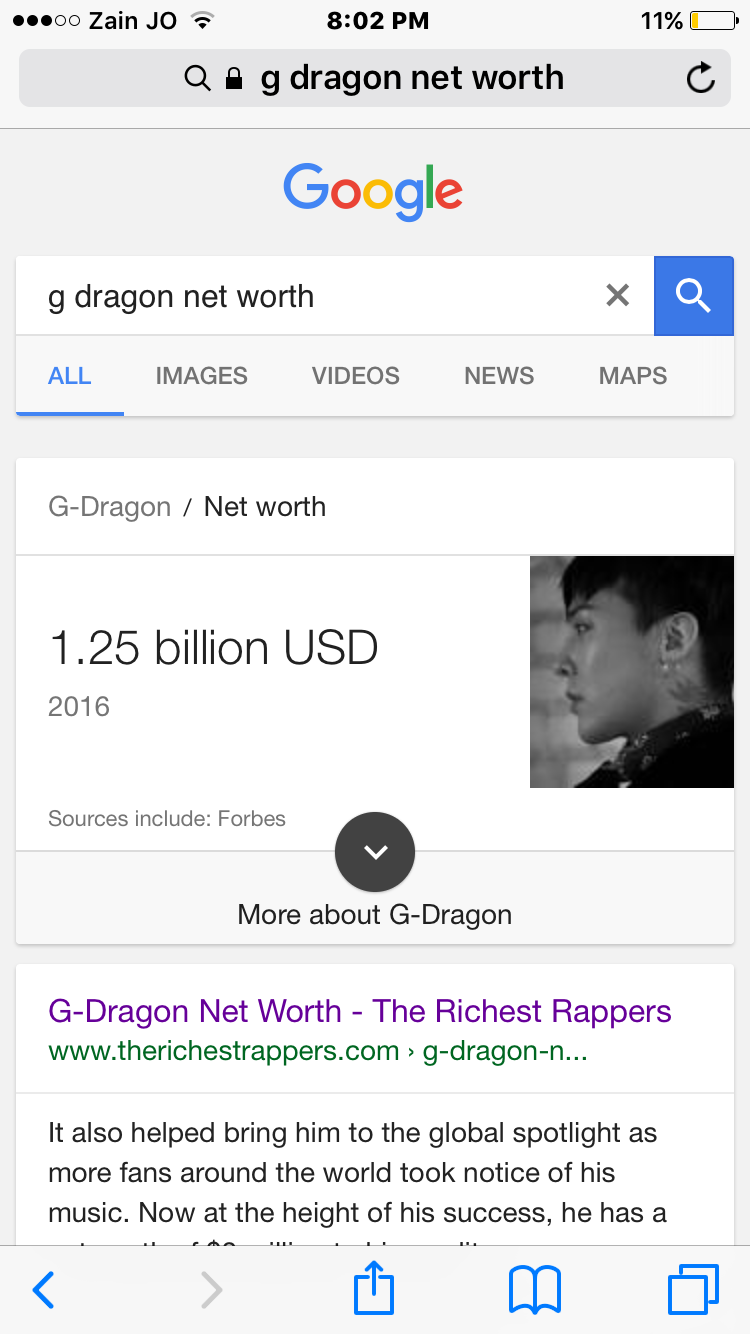This screen capture from a phone displays the net worth of G-Dragon. At the top of the screen, there are five circles, with three of them highlighted in black, followed by the text "Zane J-O." The device shows a Wi-Fi symbol with two-thirds strength, the time "8:02 PM," and an 11% battery indicator with a yellow sliver. Directly below this, there is a search box featuring a search icon, a lock symbol, and the query "G-Dragon net worth" displayed in black, along with an undo button to the right.

The Google logo, depicted in blue, red, orange, yellow, and green, appears below the search box. The search term "G-Dragon net worth" is again visible, followed by an 'X' icon to clear the query and a blue box with a white magnifying glass for initiating the search. 

Under this, options for different search categories—All, Images, Videos, Maps, and News—are listed. The "All" category is highlighted in blue, with a blue line underneath it. 

The search results display "G-Dragon net worth: 1.25 billion USD (2016), sources include Forbes" accompanied by a picture of G-Dragon to the right. 

Further down, another result is shown: "G-Dragon net worth," followed by "The Richest Rappers," in purple text linked to therichestrappers.com. The snippet reads, "It also helped bring him to the global spotlight as more fans around the world took notice of his music. Now at the height of his success he has a..."

At the very bottom of the screen are navigation icons including a back button, forward button, download button, and buttons for page management and tab switching.